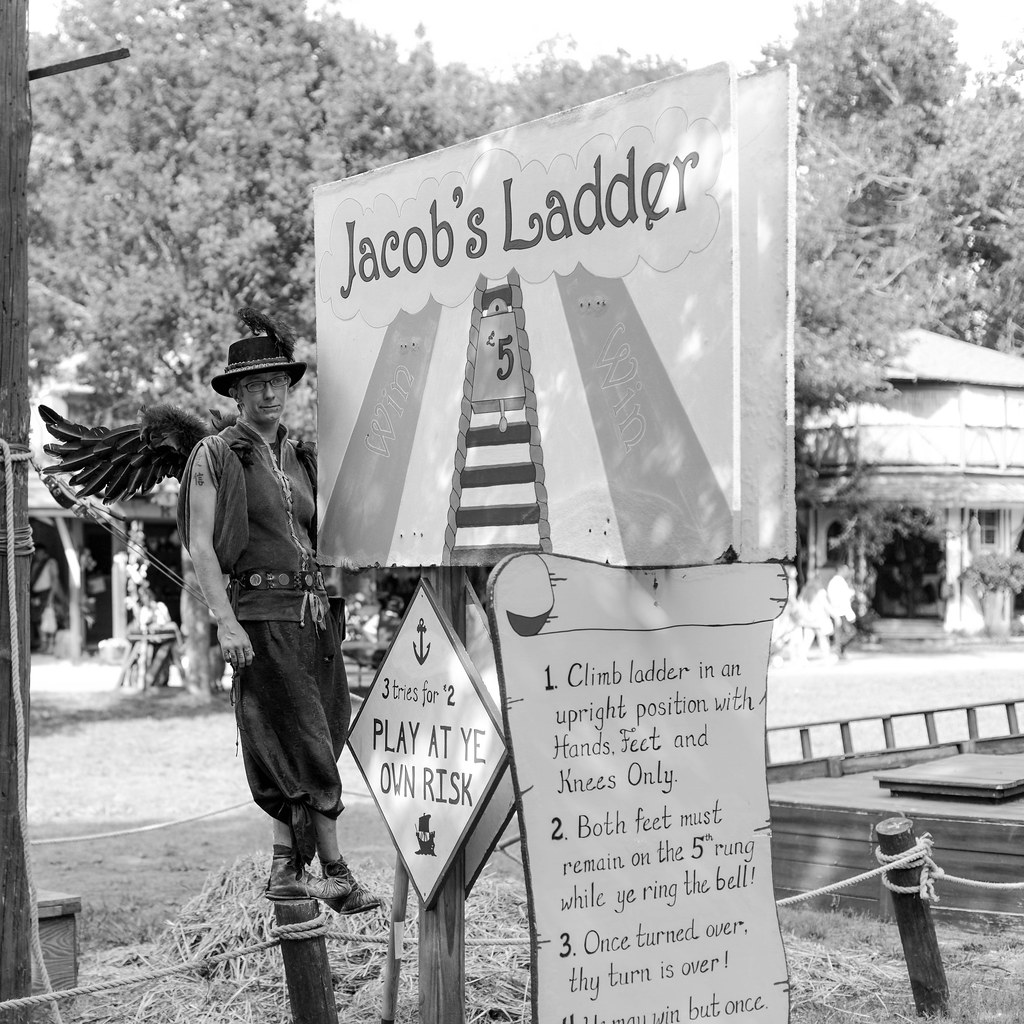This black-and-white photograph depicts a carnival or fairground setting featuring an attraction called "Jacob's Ladder." Central to the image is a large, tall sign with "Jacob's Ladder" written on it, accompanied by a picture of a ladder and a notice that reads "three tries for two dollars (or euros) – play at your own risk." To the left of the sign stands a man resembling a pirate, wearing a short top hat and medieval-like garb, complete with wings on his back. Further details of his appearance include him posing confidently next to the sign, adding a whimsical element to the scene.

The sign has additional information organized in a scroll-like design:
1. Climb the ladder in an upright position using hands, feet, and knees only.
2. Both feet must remain on the fifth rung while you ring the bell.
3. Once turned over, your turn is over.

The photograph is rich with the nostalgic atmosphere of a vintage carnival, combining elements of challenge and fantasy in its depiction.